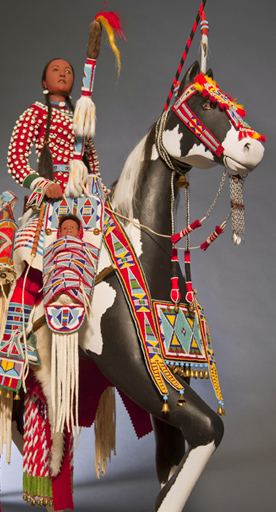The image depicts a young Native American woman with long braids, dressed in a red outfit adorned with white dots, seated atop an ornately decorated black and white horse. The woman, possibly in her 20s, holds a papoose containing her child on her right side. Both the horse and the woman are adorned with vibrant, colorful adornments featuring angular designs, including rhombuses and triangles, in hues of red, yellow, and blue. The horse’s head is also decorated with items that stick up, adding to the overall ornateness. The scene is set against a plain gray background, emphasizing the vivid colors and intricate details of the traditional Native American attire and decorations. The image, though not real, appears to represent a significant and traditional event.